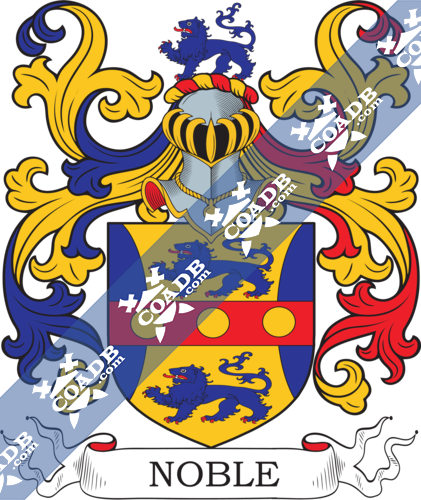This image features a detailed, computer-generated coat of arms set against a white background. Dominating the design at the center is a traditionally-shaped shield with a blue lion at the top and bottom, positioned around a vivid red stripe running horizontally across the middle. This stripe is adorned with conspicuous yellow circles. The lion figures are blue with red specks on their feet.

Beneath the shield, the word "Noble" appears prominently in black text. Crowning the shield is an ornate, silver knight's helmet with a gold faceguard and yellow accents around the eyes. Protruding from the helmet are elaborate, hair-like decorations that are yellow and blue on the left, and yellow and red on the right. Topping the helmet, there is another blue lion figure. Diagonally traversing the image, a recurring strip reads "COADB.com," adding a modern touch to this heraldic design.